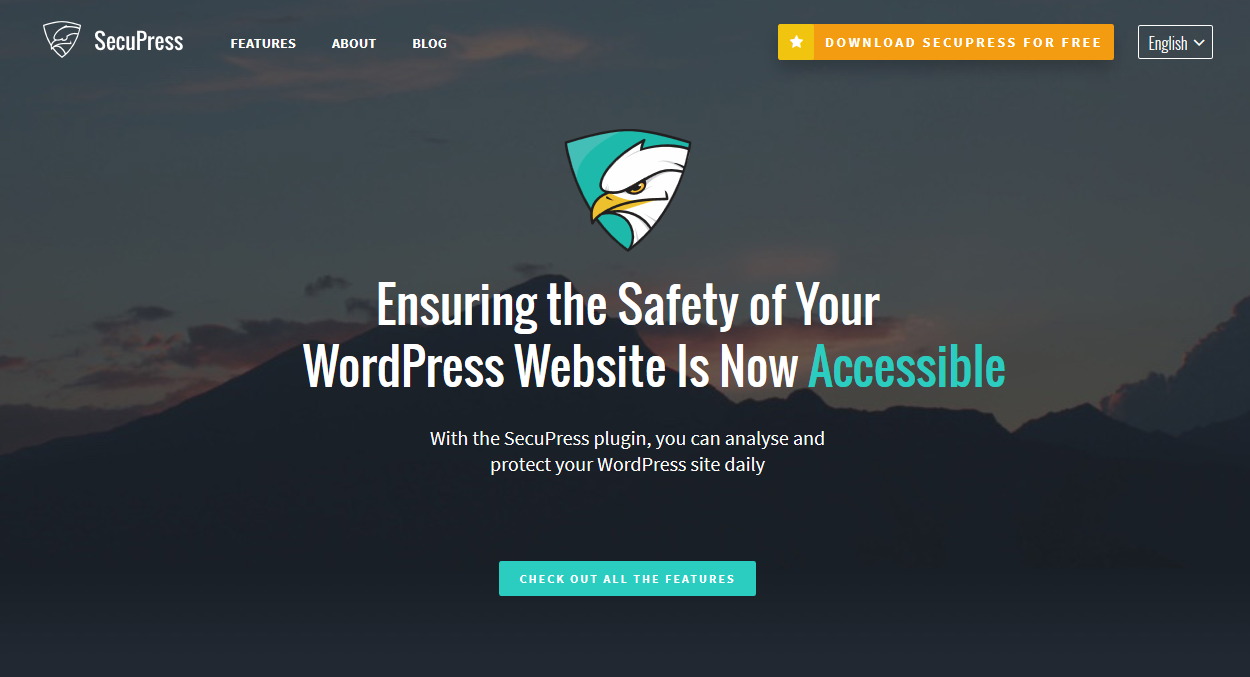The homepage of SecurePress features a navigation menu at the top with options for 'Features,' 'About,' and 'Blog.' To the right, there is a prominent orange button labeled 'Download SecurityPress for Free.' Adjacent to this button is a language selection dropdown menu displaying 'English' with a downward-facing arrow.

The background of the page is a dark, serene landscape of mountains against a sunset sky. The clouds are tinged with shades of pink and purple, providing a striking contrast. Central to the design is a drawn emblem of an eagle within a shield, symbolizing vigilance and protection.

Below the emblem is the tagline, 'Ensuring the Safety of Your WordPress Website is Now Accessible.' This is followed by an explanation: 'With the SecurityPress plugin, you can analyze and protect your WordPress site daily.' At the bottom of the page, there's an aqua-colored button inviting users to 'Check Out All the Features.' The overall design is geared towards highlighting the plugin’s capabilities in a visually engaging and informative manner.